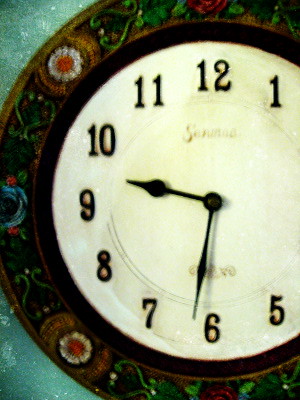A close-up of a vintage ceramic clock face is prominently displayed. The clock features a classic white round face, slightly stained with age, and marked with numbers 1 through 12 in a traditional font. The center of the clock showcases a small pinstripe circle, accompanied by a logo beginning with the letter 'S.' Two elegantly designed black metal hands extend across the face; the hour hand is shaped like a spade, while the minute hand forms an elongated diamond. Encircling the clock is a black frame embellished with intricate embroidery, depicting white flowers and a mix of green, blue, and red floral patterns. The ornate frame slightly extends beyond the clock, adding a touch of ornate craftsmanship. Beyond this embroidered frame, two darker turquoise blue sections appear in the upper left and lower left corners, providing a striking contrast and completing the elegant and detailed design of the clock.